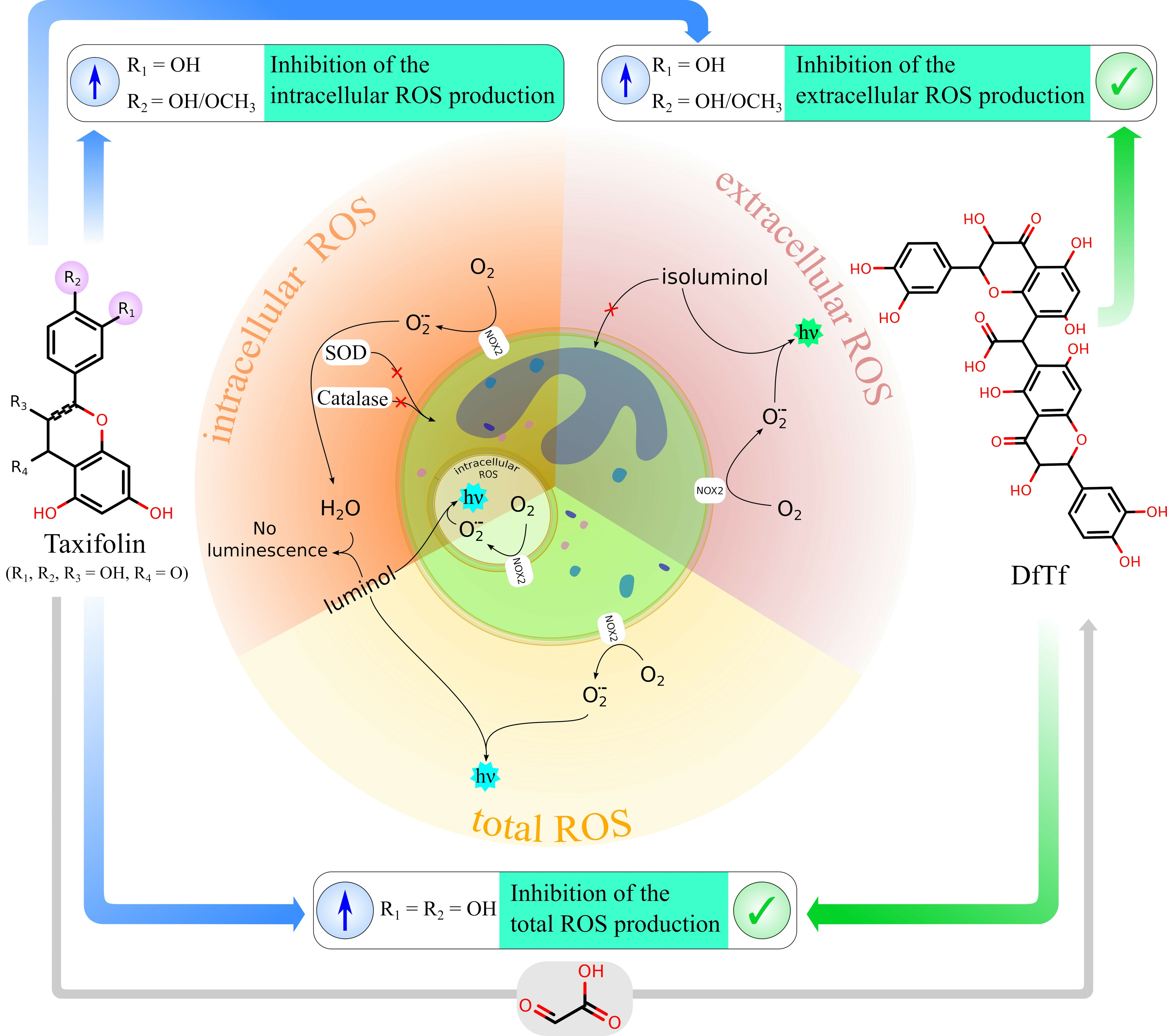The detailed and comprehensive image is a colorful digital chart illustrating molecular designs and cellular processes related to ROS (reactive oxygen species). Central to the chart is a green cell model with detailed annotations. The image is segmented into different areas showing intracellular ROS at the bottom, extracellular ROS on the right, and overall ROS indicators. Various color-coded arrows (red, yellow, green, blue, orange, pink) direct attention to specific pathways and molecules such as taxifolin and DFTF, highlighting the mechanisms of ROS inhibition and production. The chart uses a Times New Roman Serif font for all its text, making it clear and legible. Additional elements include labels like O2 and H2O, showing the involvement of different molecular species. The background of the chart is predominantly white, providing a clean canvas for this highly detailed scientific diagram.